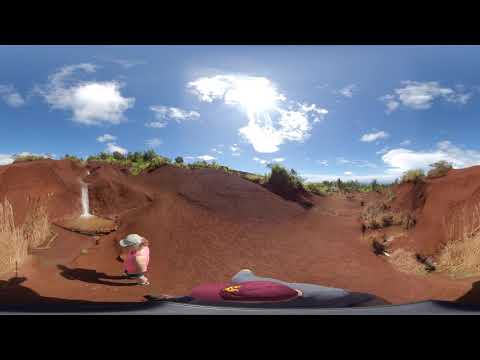The image portrays a sunlit outdoor scene featuring expansive, reddish-brown hills and a touch of desert-like aridity. At the top, a blue sky populated with puffy white clouds—particularly bright and prominent in the center—stretches across. Green grass patches and scattered green trees are visible, including some areas of dry, dead grass near the bottom right. A woman in a pink jacket, dark pants, and a white cap stands on the left, her shadow cast against the hills. Notably, there's a suggestion of a small waterfall on the left side, surrounded by shrubs and small bushes. The landscape, generally a mix of muddy and dry terrains, includes visible pathways winding through rolling hills, resembling a small, verdant valley interspersed with reddish-brown earth.